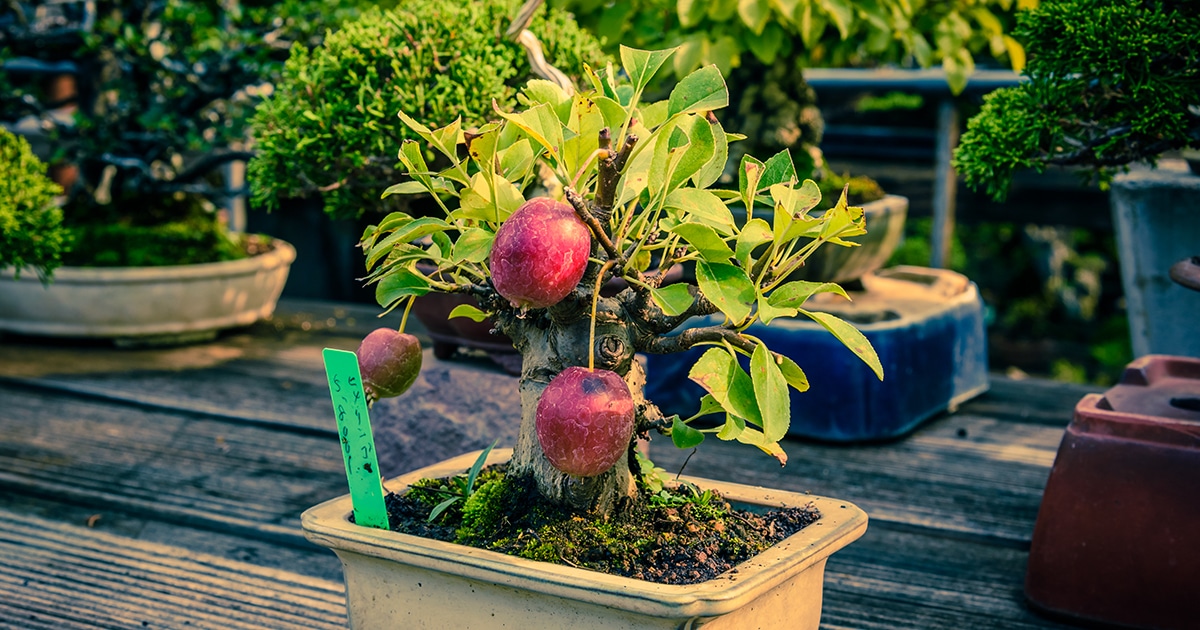In a sunlit garden scene, a collection of small trees and plants is showcased on a light tan wooden porch. The centerpiece is a rectangular, light tan planter box with a flared lip, filled with dark brown soil and green, grassy moss at the base. Emerging from the soil is a small tree adorned with vibrant green leaves and bearing red fruit that looks like cherries or tiny apples, with some of the fruit appearing frozen, encrusted with a thin layer of ice and delicate icicles. Surrounding this central planter are various vessels in different shapes and colors, including round, rectangular, blue, and brown pots, each containing diverse bonsai trees and small plants. The entire arrangement rests on a patterned garden platform, enhancing the cozy and natural aesthetic of the porch.